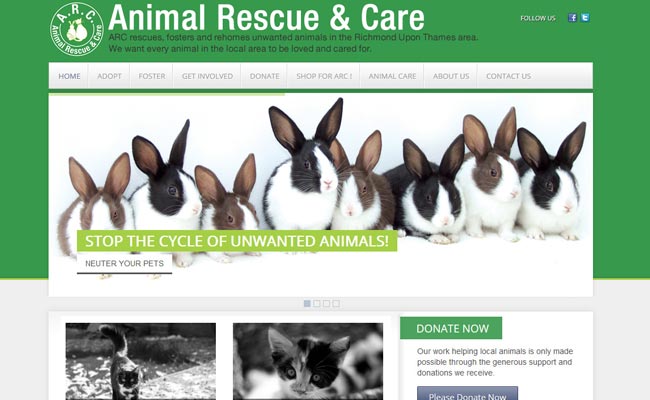For the AHRQ (Animal Rescue and Care) organization, the image features a vibrant green background accented by crisp white text. Central to the design is an emblem: a circular white logo containing silhouettes of various animals. Around this emblem, the organization's name, "AHRQ," is thoughtfully curved, emphasizing its mission: "AHRQ rescues, fosters, and rehomes unwanted animals in the Richmond-Upon-Thames area. We strive for every animal in our community to be cherished and well-cared for."

Prominently displayed in white, capitalized text against the green backdrop is a call to action: "Follow Us." Accompanying this are recognizable social media icons—a white Facebook "F" within a blue box and a Twitter bird emblem, symbolizing their presence on these platforms.

Below this section, the navigation menu offers various options: Home, Adopt, Foster, Get Involved, Donate, Shop for AHRQ, Animal Care, About Us, and Contact Us. 

The main visual features eight bunnies: two tan, four black and white, and three brown and white, accompanied by an urgent message in a green rectangular banner with bold, capitalized white text: "STOP THE CYCLE OF UNWANTED ANIMALS!" Beneath this message, a directive in a white box with black, capitalized text, reads, "NEUTER YOUR PETS," emphasized by a black bar underneath it. Four squares follow, with the first filled and the remaining three empty.

Additional images depict cats with a gray background and white framing. One black cat with a white chest is pictured outdoors on a stoop amidst fallen leaves, while a black, white, and brown cat reclines indoors, likely on a couch or bed.

A prominent white rectangle houses a green "DONATE NOW" button with white capitalized text, underscoring the message: "Our work helping local animals is only made possible through the generous support and donations we receive." This is complemented by an additional blue "PLEASE DONATE NOW" button, also in white text.